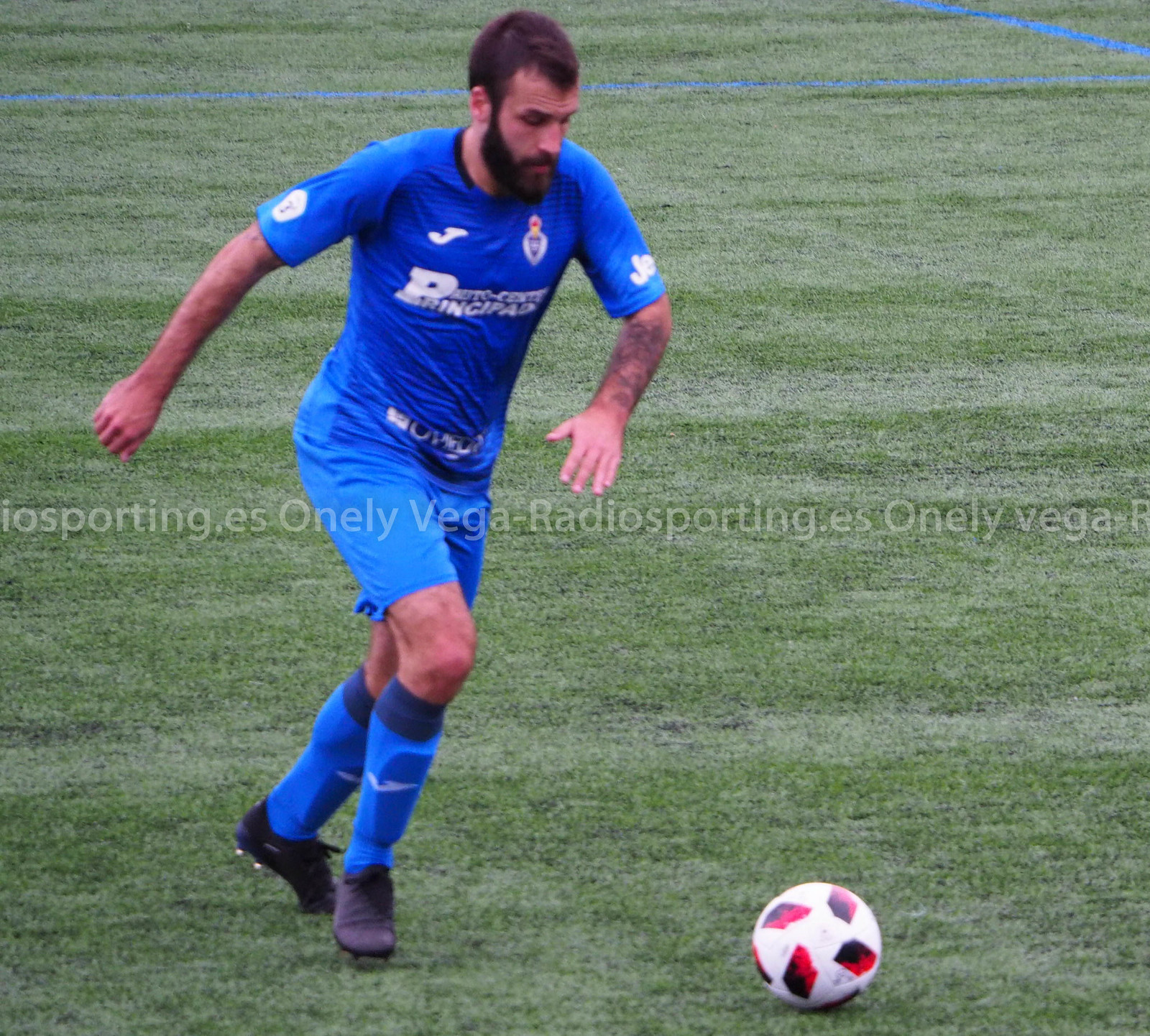A photo captures a soccer player on a grassy field marked with blue lines in the background. The player, a Caucasian man with short black hair and a short black beard, is seen running towards a soccer ball that is white, black, and red, positioned at the bottom edge of the picture. He's wearing a blue outfit consisting of a t-shirt with white text and logos on the sleeve and front, blue shorts, knee-high blue socks, and black soccer shoes. The jersey displays the words "Swoom in. Principad Auto Center" and has a logo resembling a "J" on his right lapel, possibly indicating "JEEP" on his left shoulder. There is also a visible watermark over the image that reads "osporting.es onely vega-radiosporting.es onely vega." The field is green, and the overcast sky results in the absence of shadows, highlighting the action-focused moment of the player about to kick the ball.